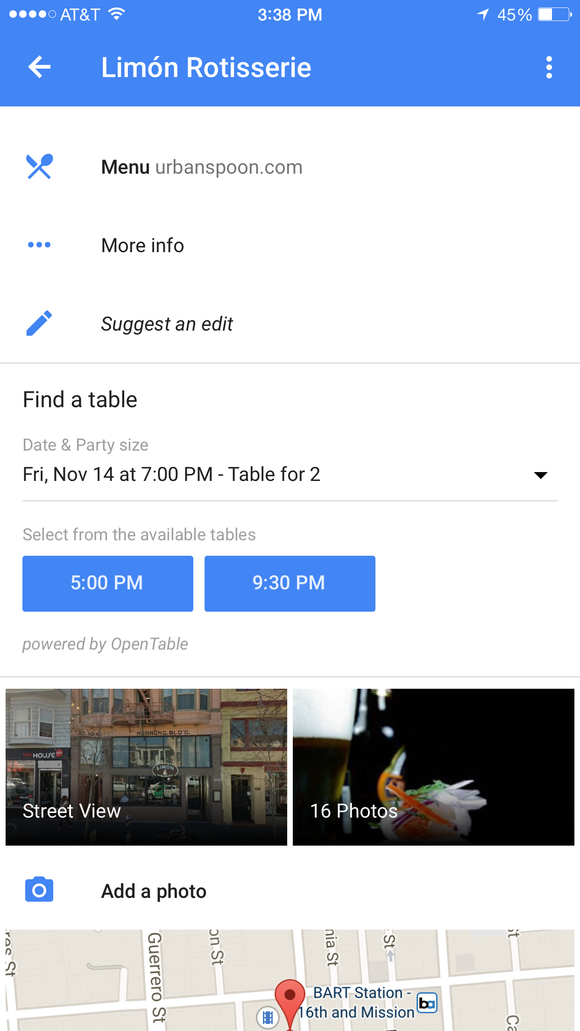This image is a detailed screenshot from a smartphone showing an online reservation page for Limon Rotisserie, a restaurant. 

At the top, the smartphone's status bar features a blue header. The upper-left corner displays four white dots symbolizing a strong, but not full wireless signal, accompanied by the text "AT&T." Near the center, the time is displayed in white font as 3:38 p.m. On the far right, the battery icon indicates a 45% charge.

Below the status bar, the webpage background is white with black text prominently displaying "Limon Rotisserie." The menu details are labeled in black font, followed by "UrbanSpoon.com" in gray. Additional options are labeled beneath, including "More info," "Suggest an edit," and "Find a table."

The reservation section indicates a selected date and party size: Friday, November 14th at 7 p.m. for two people. Below this, two blue rectangles (matching the header color) present alternative reservation times at 5 p.m. and 9:30 p.m. A light gray text at the bottom reads "Powered by OpenTable," showcasing the platform facilitating the reservation.

The lower portion of the screenshot includes a street view photo of the restaurant and a clickable link labeled "16 photos" to view more images. Additionally, a partial Google map with a location marker is visible, identifying the nearby BART station, suggesting the restaurant is located in the San Francisco Bay Area.